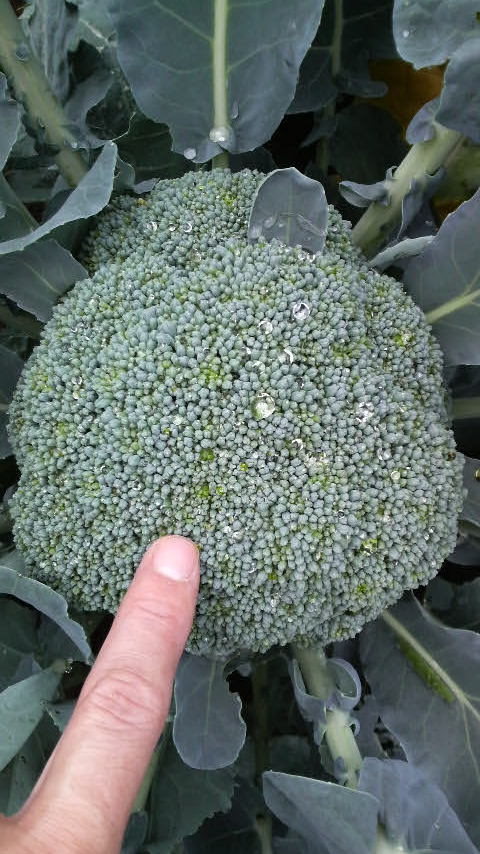This close-up photograph captures a large, vibrant head of broccoli growing in a garden on a sunny day. The central focus is the broccoli head, which is light green with vibrant, almost lime-green tones, adorned with small water droplets that glisten, suggesting it's either freshly watered or has dew on it. The surrounding leaves are a lush, vibrant green with visible light green veins, though some leaves exhibit signs of damage, either from pests or natural wilting. Among these leaves, a small green worm can be seen, likely the culprit behind the damage. Notably, a human hand enters the frame from the bottom left corner, with a medium skin-toned pointer finger touching the broccoli, emphasizing the considerable size of the head. A small fallen leaf perches atop the broccoli, reaching upwards. This comprehensive image showcases both the beauty and the natural imperfections of a thriving garden vegetable.